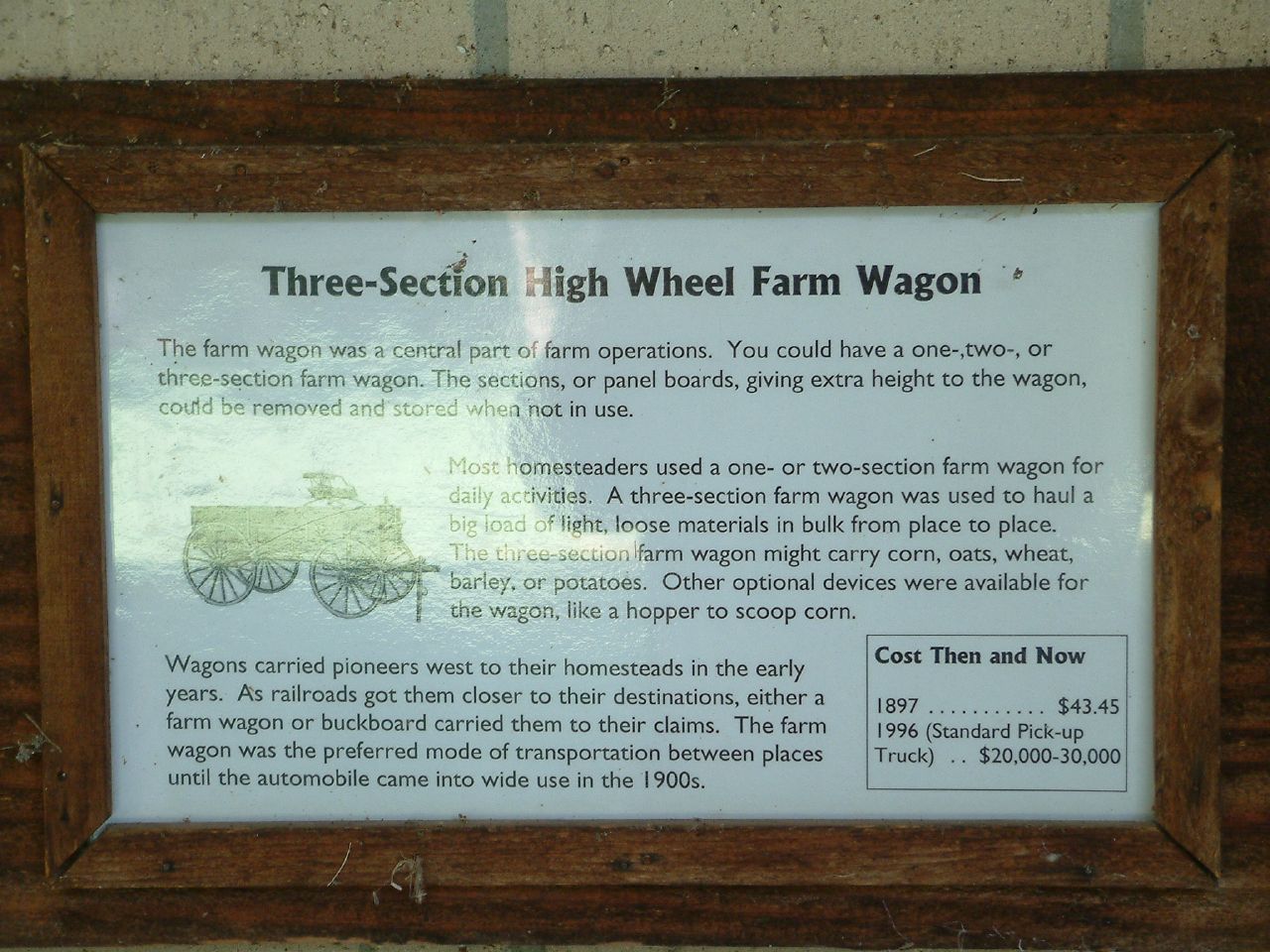The image is of a wide rectangular sign mounted on a light tan brick wall, visible only at the top of the image, with bricks separated by thin rows of gray cement. The sign is encased in a dark brown wooden frame that is slightly lighter on the inside. It contains a laminanted white piece of paper with text written in thick black font at the top that reads "Three Section High Wheel Farm Wagon." The sign describes the farm wagon as a central part of farm operations, indicating that it could be configured with one, two, or three sections, with panel boards that could be removed and stored when not in use. The text explains that a one or two section wagon was typically used for daily activities, while a three section wagon was used for hauling bulk materials such as corn, oats, wheat, barley, or potatoes. It also mentions that wagons played a crucial role in transporting pioneers to their homesteads. A black and white drawing of an old-fashioned wagon is featured on the left side of the sign. Additionally, it highlights the historical costs of the wagon—$43.45 in 1897 and the equivalent of $20,000 to $30,000 for a standard pickup truck in 1996.